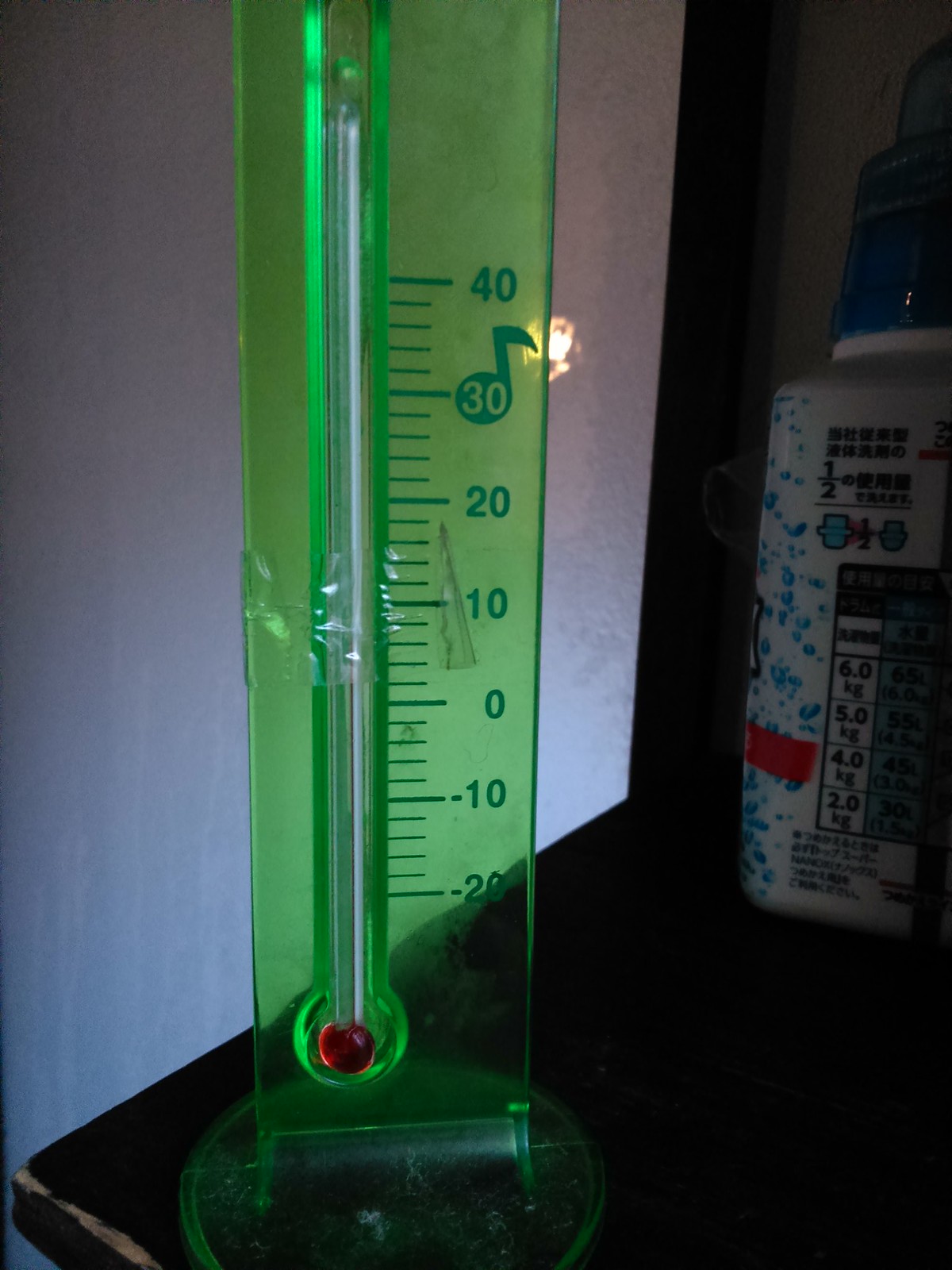This image features a lime green, see-through plastic thermometer, set indoors on a worn brown table. The thermometer, with a round base, is positioned near the edge of the table, which shows signs of use, especially on the corners. The thermometer's scale runs from the top, starting at 40 degrees, down through 30, 20, 10, zero, and into the negatives: -10 and -20 degrees. Notably, the number 30 is styled as a musical note. The scale is marked along the right side of the thermometer. Centrally on the left side, the mercury column is visible, and a piece of tape is affixed over the plastic near the 10-degree mark. At the bottom of the thermometer, a red circle indicates the lower end of the scale, where the tube containing the temperature-sensitive liquid is securely held in place.